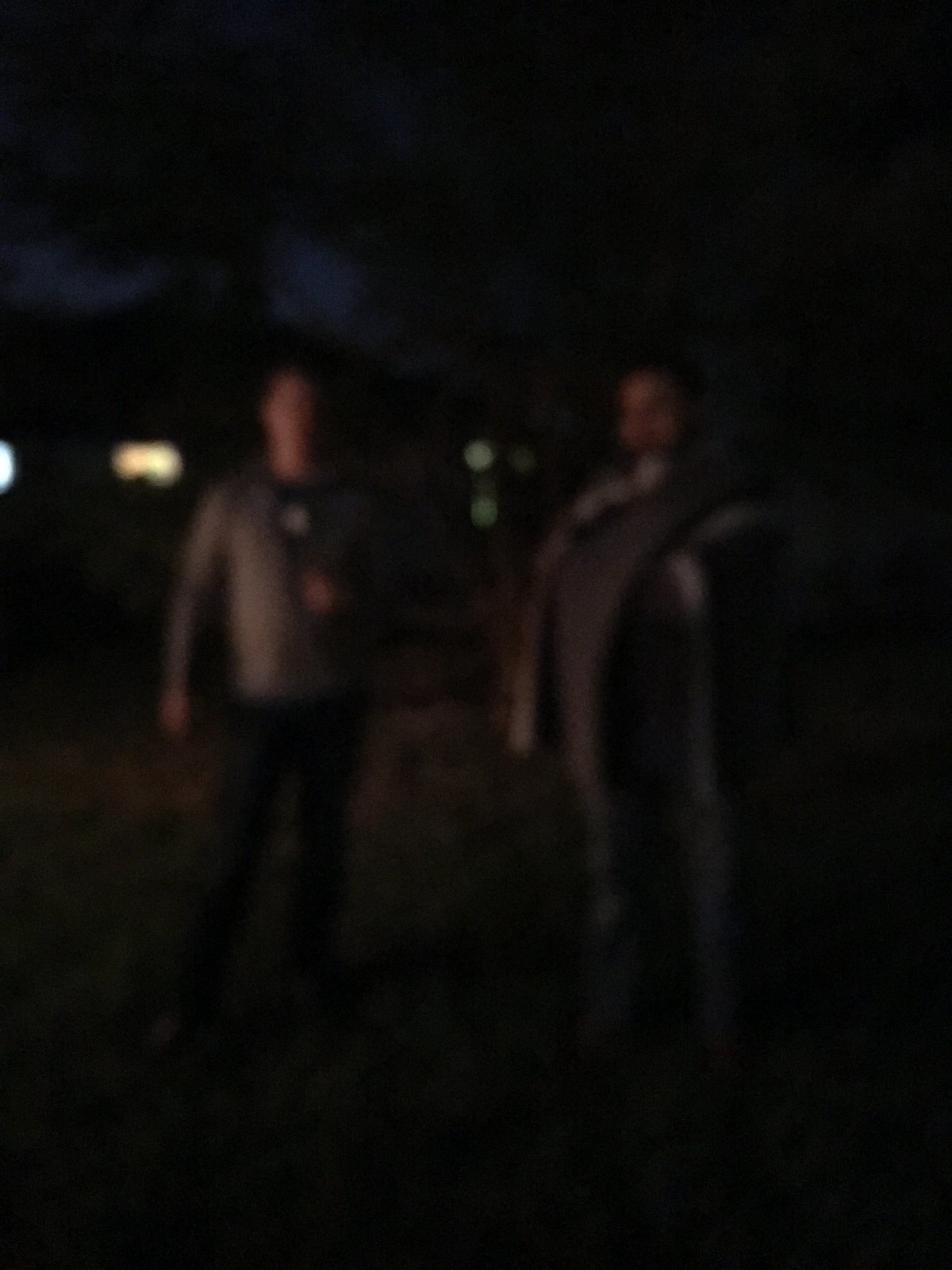The photograph is a very dark and blurry capture of two men standing outside at night, taken with a low-quality camera or cell phone. The night sky appears dark blue in one section above the man on the left, possibly indicating some sky peeking through trees. The surroundings include a mix of green and brown grass, and there might be a tree overhead. In the distant background, there are lights that could be from a car or a one-story house with a light on.

In the center, the focus is on two men. The man on the left, possibly Caucasian with brown hair, is wearing black pants and a gray long-sleeved shirt. His right arm hangs down by his side, while his left arm appears to be bent at the elbow, possibly holding an item. The man on the right, larger in build, is wearing dark-colored long pants. He has something hanging from his neck area, which might be a scarf or a blanket. The poor lighting and blurred image obscure many details, including their feet and finer facial features. Only their chest areas and parts of their faces are somewhat discernible.